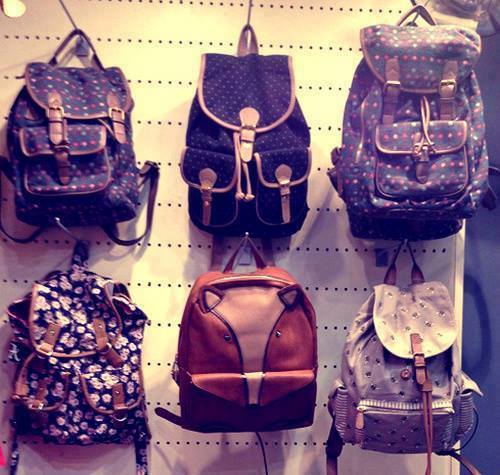The image displays six small, vintage-style backpacks hanging on a white pegboard wall, which has numerous vertical rows of holes and metal hooks. Starting from the top row, the first and third backpacks are identical, featuring a dark navy blue or black background with red, white, and blue polka dots, brown leather straps, piping, and buckles. The first backpack also has a front pocket and two buckles on the top lid. Sandwiched between these two, the central backpack is darker blue with lighter blue dots, equipped with brown edging around the pockets —two in the front and one on top— and has tassel strings hanging down.

On the bottom row, the first backpack from the left is blue with a floral pattern, having three pouches with buckles. The central backpack stands out with an animal-face design, possibly a fox or anteater, showcasing small ears and eyes. It's primarily brown leather with a lighter brown section down the center and a possible zipper on the front. The final backpack on the right features a white background with a black floral pattern resembling daisies or possibly insects like ladybugs or bees. It has a zippered pocket at the bottom and side pockets, all complemented by brown leather piping and buckles.

Overall, the display presents a somewhat muted and traditional aesthetic, likely aimed at a younger female demographic, with all backpacks sharing brown leather straps and a classic design reminiscent of old-school backpacks or purses.